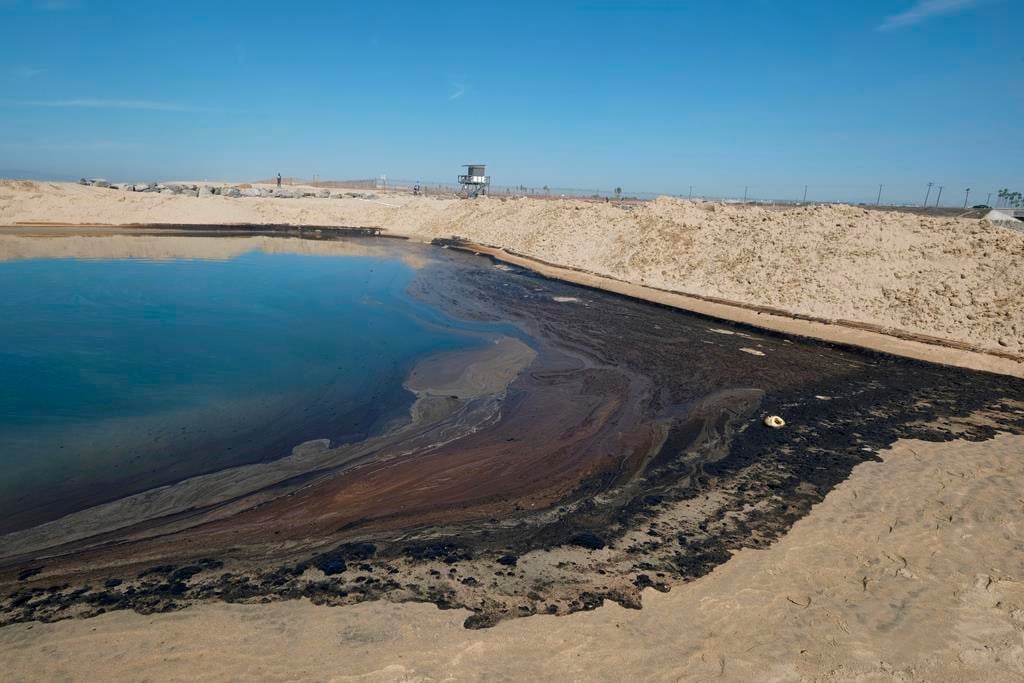The image captures a beach scene under a clear blue sky, defined by an expansive view of water and sandy soil stretching across the bottom right side of the frame. Prominently featured is a large, square pit filled with black, reflective liquid that resembles oil, with brownish-gray streaks running around its edges. This pit is surrounded by sandy dunes, as if the sand has been pushed aside to form a barrier. Mixed into the dark liquid are patches of sand, witnessing the merging of natural and contaminated elements. In the foreground, a small white shell contrasts sharply with the blackened sand. Far in the distance, a wooden lifeguard watchtower stands against the horizon, hinting at efforts to monitor and protect the area. The overall scene reflects the impact of a man-made disaster on an otherwise serene coastal landscape, with a clear demarcation between the polluted section and the untouched sand beyond a small protective hill.